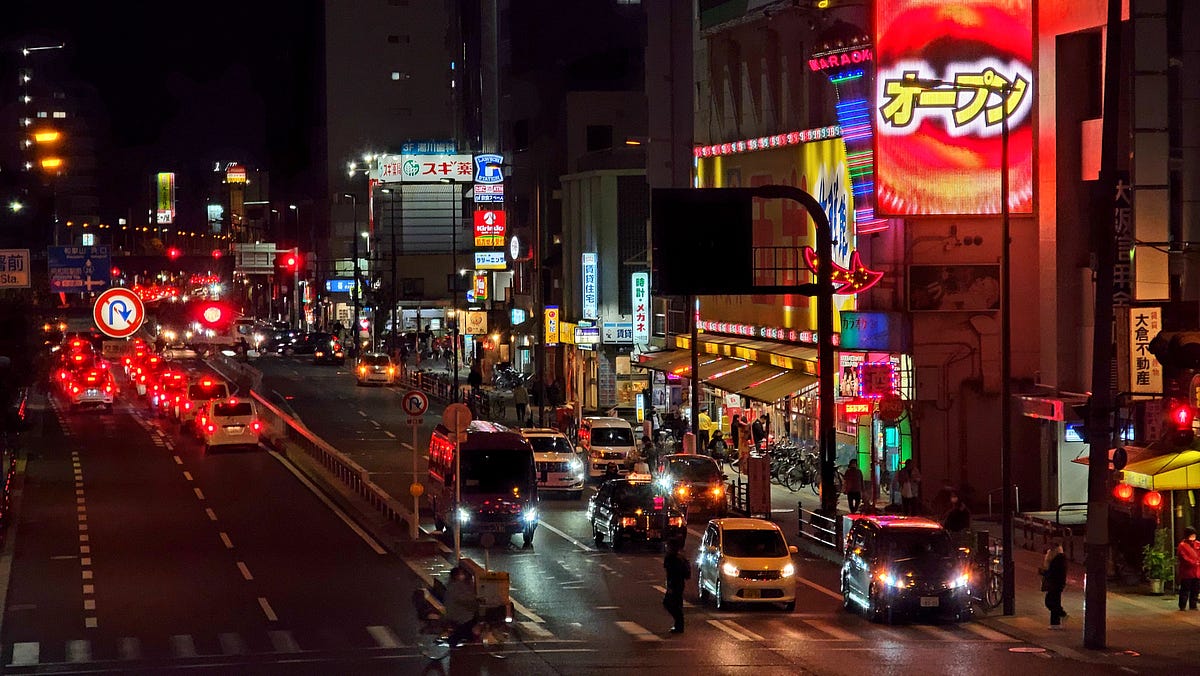The image captures a bustling Japanese downtown area at night, viewed from a high angle, perhaps from a balcony or parking garage. The scene is lively with numerous colorful neon signs in reds, yellows, and blues, advertising various businesses including restaurants and karaoke bars. The street is alive with activity: many pedestrians crossing the sidewalks, and a significant number of cars traveling along what appears to be a four-lane road cutting diagonally from the bottom to the left side of the image. The road is busy, with taillights illuminating the left lanes and headlights the right lanes, but it's not gridlocked. The buildings on the right side are multi-story and made of concrete, adorned with a multitude of brightly lit signs, one of which is a prominent red square sign featuring yellow Japanese characters. An overhang and a couple of parked bicycles are also visible. The sidewalk continues parallel to the roadway, extending along the vibrant strip of storefronts and other lit signs, indicating a thriving nightlife in this part of the city.